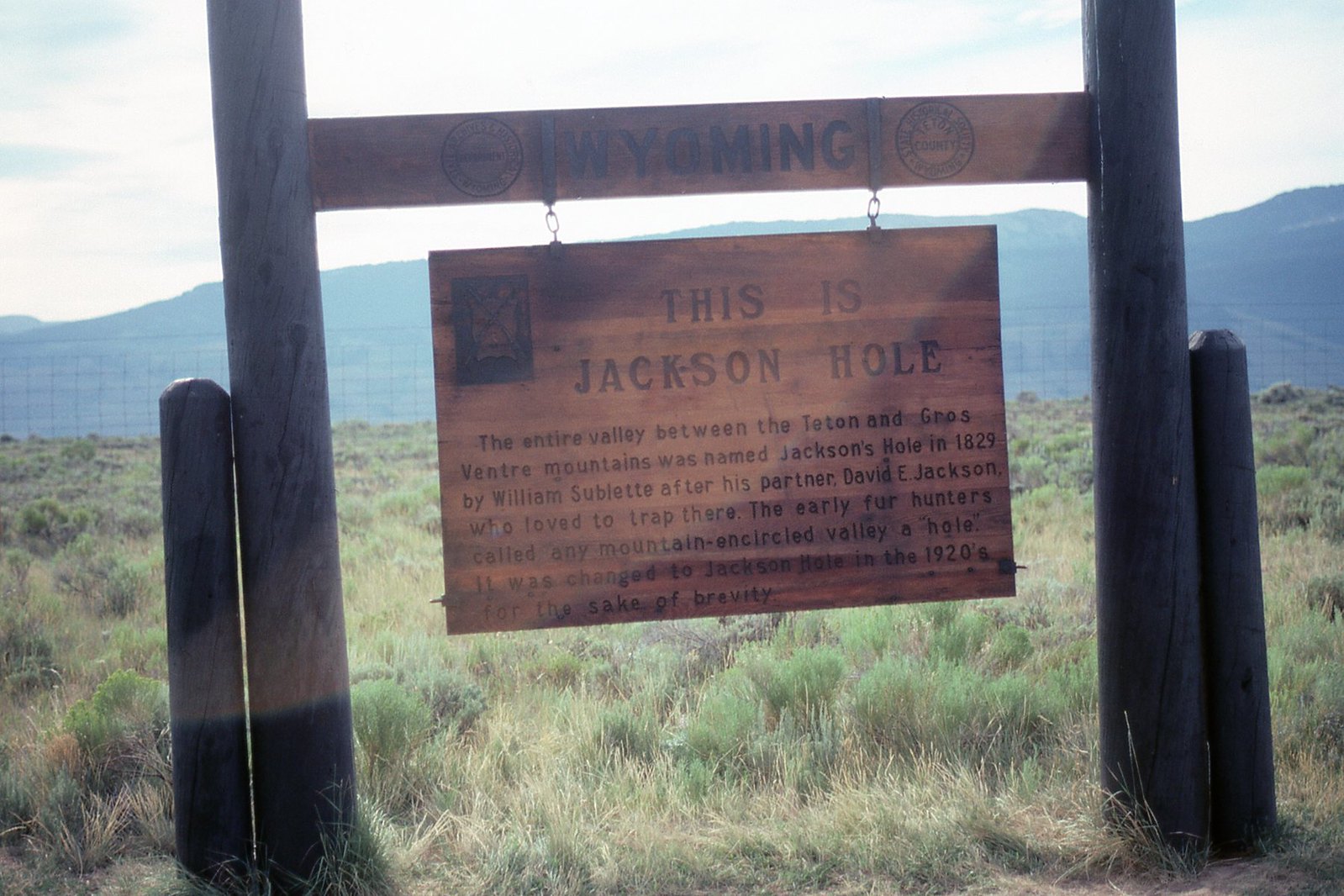The image depicts a large wooden sign within a natural reservation or national park, set against a grassy landscape with small bushes and a faint wire fence in the background. The sign, supported by two thick wooden posts and flanked by two smaller posts, bears the name "Wyoming" burnt into a horizontal plank. Hanging from this plank by chains, another wooden sign reads: "This is Jackson Hole. The entire valley between the Teton and the Grosse Ventre Mountains was named Jackson's Hole in 1829 by William Sublet after his partner, David E. Jackson, who loved to trap there. Early fur hunters called any mountain in Circle Valley a hole. It was changed to Jackson Hole in the 1920s for the sake of brevity." Behind the sign, low mountains or hills emerge faintly in the distance under a mostly white, overcast sky with hints of blue. The overgrown grass and the scattered small bushes emphasize the natural, untamed beauty of the area.